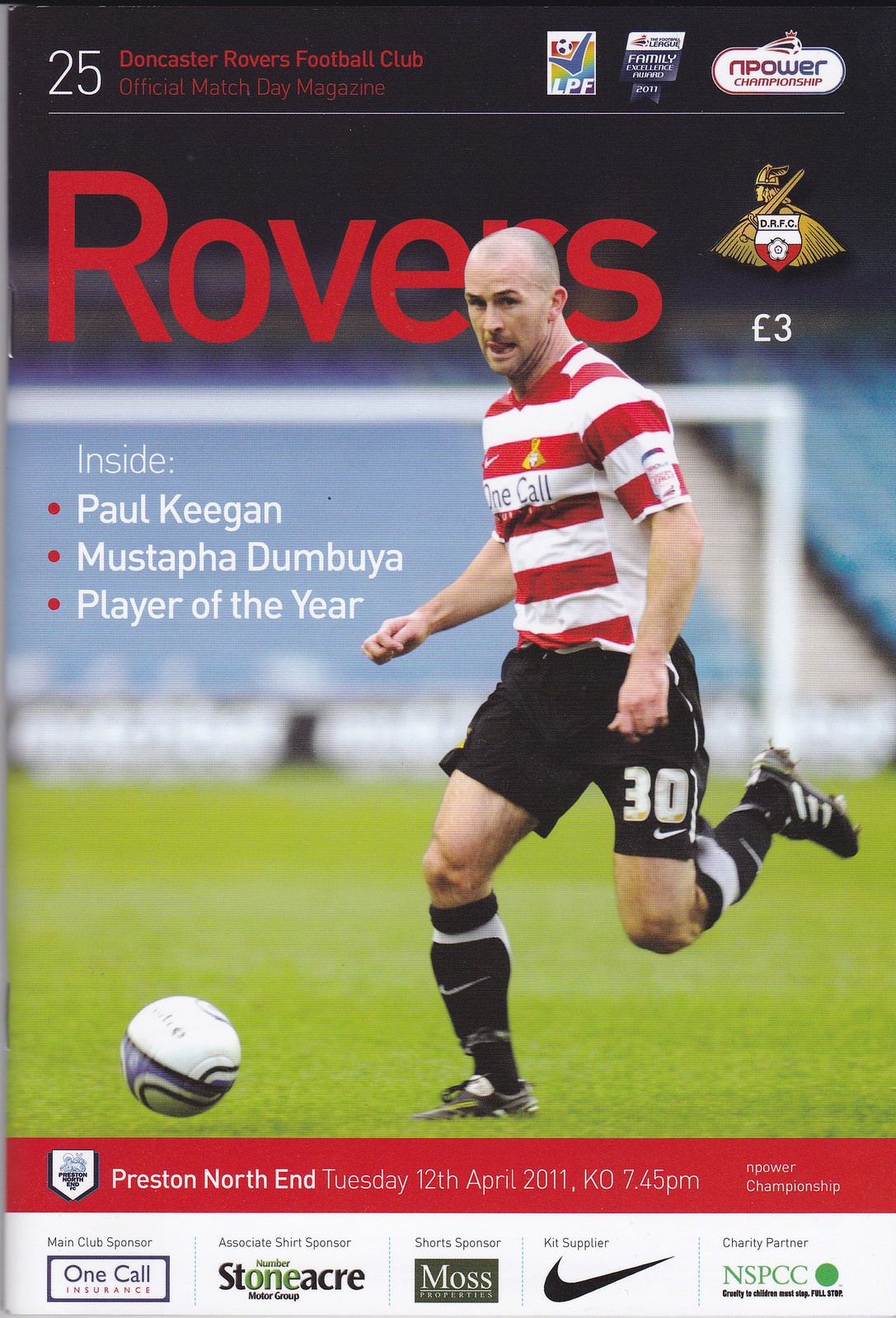The cover of the Doncaster Rovers Football Club Official Match Day Magazine prominently features a side-view photograph of a soccer player wearing the team's white and red striped shirt with the number 30 on his black shorts and black Nike shin guards. The player is poised to kick a soccer ball, set against the backdrop of a soccer field with an out-of-focus goal and blue seats. The top of the cover reads "White 25" followed by "Doncaster Rovers Football Club Official Match Day Magazine" in red. Across the image, the title "Rovers" is displayed in bold red, partially obscured by the player's head. In the left corner, text in white highlights "Inside: Paul Keegan, Mustapha Dumbuya, Player of the Year." The bottom section of the cover, marked by a red banner, details an upcoming match against Preston North End on Tuesday, 12th April 2011, at 7:45 PM, along with sponsor information including One Call Insurance, Stoneacre, and the charity partner NSPCC.